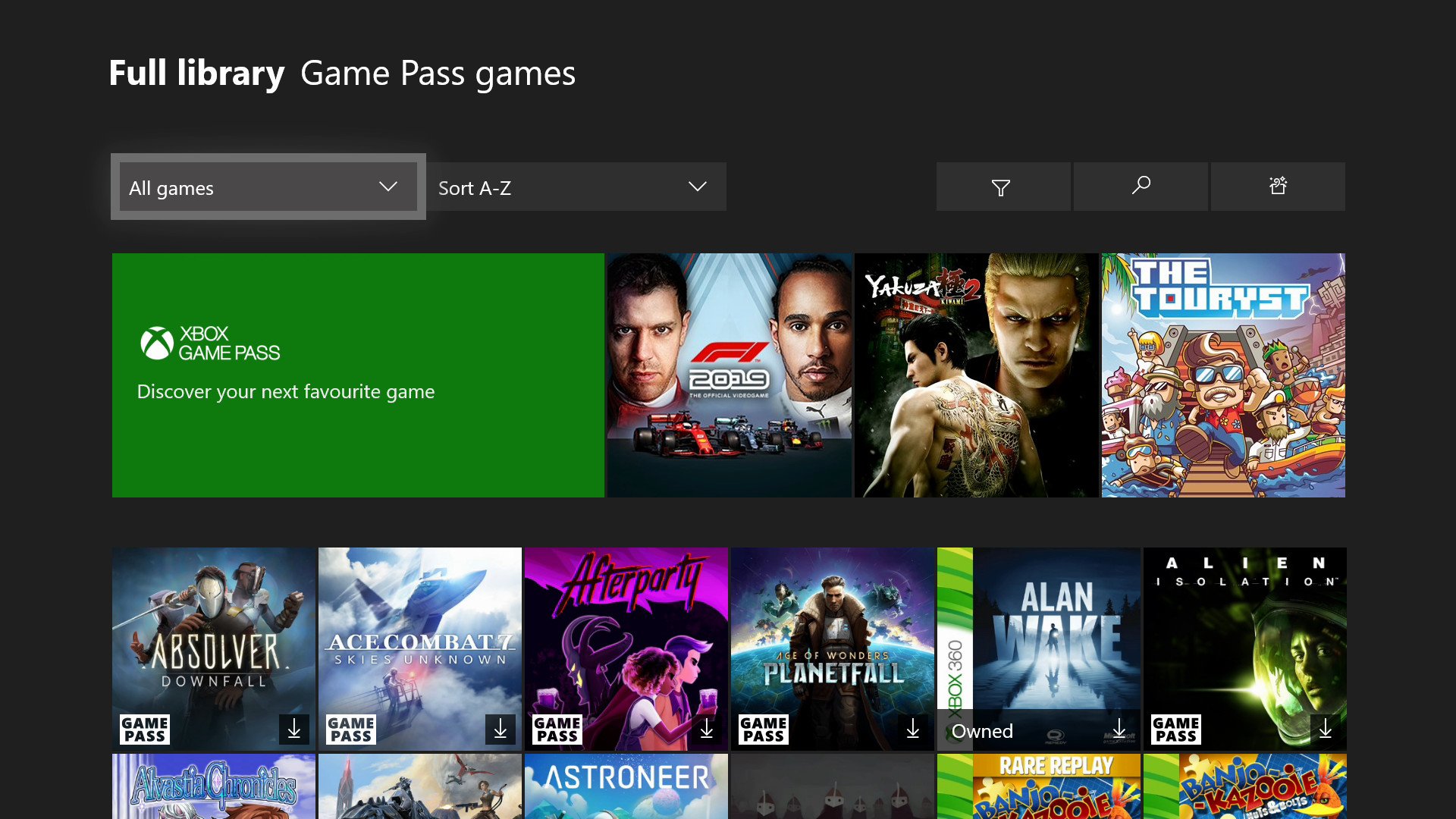The website features a sleek, black background design with an intuitive layout for users to explore Game Pass offerings. At the top of the page, a prominent header reads "Full Library of Game Pass Games". Underneath this, there is a user-friendly search bar labeled "All Games", accompanied by a sort filter labeled "A to Z". Both options feature drop-down menus for easy navigation. 

Adjacent to the search bar, a filter button allows users to refine their game search criteria, while a magnifying glass icon offers a direct search function. Nestled next to these is a small box icon resembling a gift, possibly indicating options for gift cards or special offers.

Below these navigation tools is a striking green banner with the text "Xbox Game Pass – Discover Your Next Favorite Game". This section highlights various games available on the platform. Featured titles include:

1. A 2019 racing game.
2. Yakuza, showcasing a character with an elaborate back tattoo.
3. The Touryst, depicting cartoon characters enjoying water activities.
4. Absolver, featuring a masked character wielding a sword.
5. Ace Combat, illustrating an intense aerial combat scene.
6. Afterparty, with a distinct manga-style design.
7. Planetfall, Alan Wake, and Alien, adding variety with their unique art and gameplay styles.

Overall, the design facilitates a seamless browsing experience, encouraging users to discover a diverse range of games.